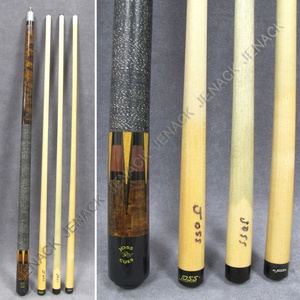This composite image features two photographs of pool cues arranged side by side. On the left, a more distant shot shows four pool cues: three with light, yellowish wooden shafts and small black caps at their bases, each elegantly inscribed with the name "Joss" in brown vertical lettering. The fourth cue stands out with its intricate design, featuring a black base transitioning into a burl wood segment, adorned with patterned black and white dots and thin, orangish triangles. Its shaft is silver, culminating in a white tip. On the right, a close-up image highlights the bases of these cues. Here, the distinctly crafted cue reveals additional details of its inlaid design, with dark brown wood, red, and yellow triangular patterns extending toward the base, also marked "Joss Cues" near a black band. Both images are set against a plain, gray backdrop, and a watermark reading "Jenack" can be seen across the photos.